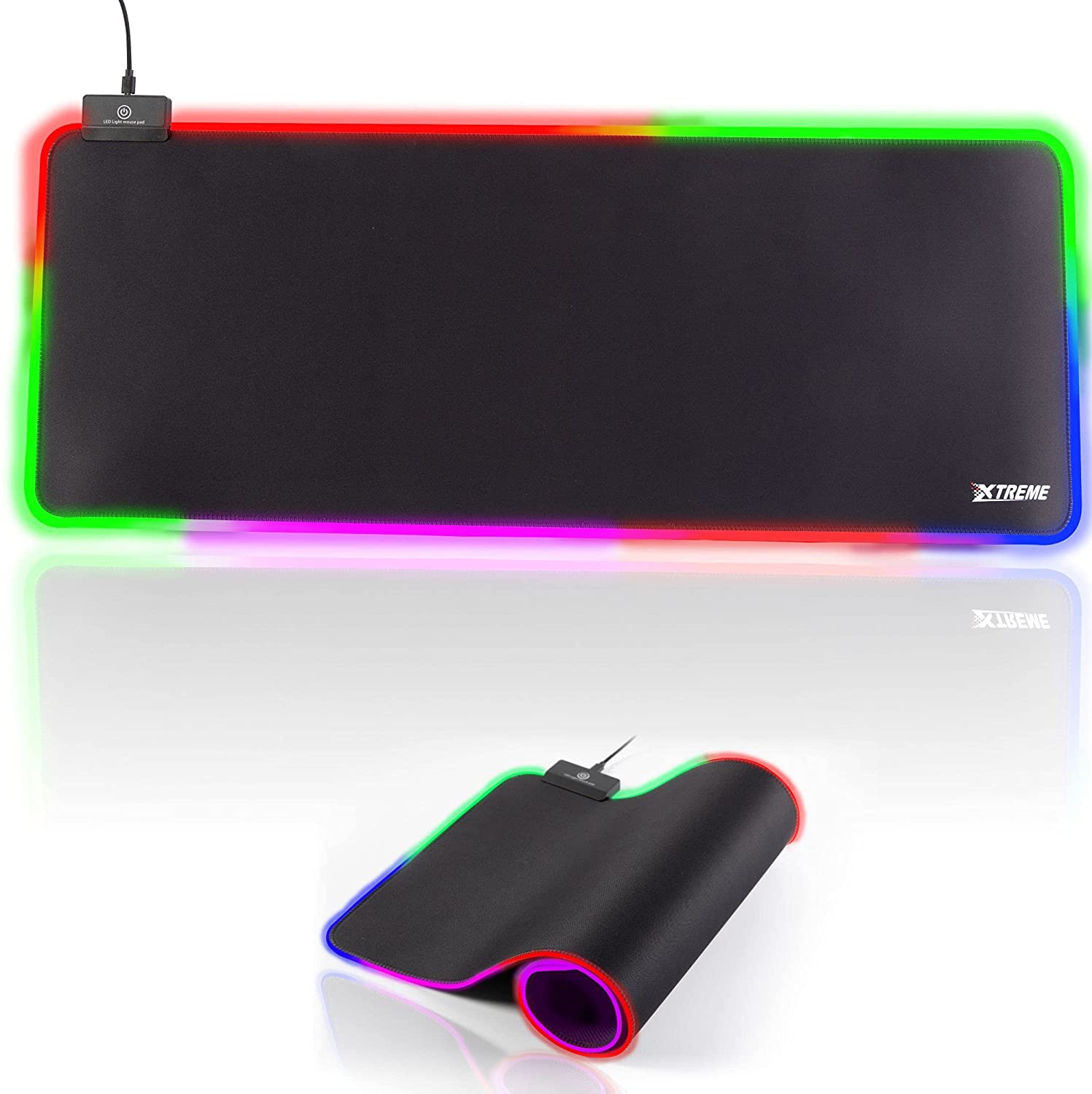The image depicts a black rectangular electronic device, possibly a synthetic foam or fabric material, with a long screen resembling a phone laid horizontally at the top. In the top left corner, a small black attachment with a wire and antenna is connected. The device's perimeter features a vivid multicolored border: red starting from the top left corner, transitioning to green at the top right, blue around the bottom right, purple and red across the bottom, and finally green rounding the bottom left corner to meet the red again. The lower section of the image includes another angled view of the device, slightly rolled to reveal a central cylindrical shape. Additionally, the bottom right corner of the device displays the brand name "XTREME" in white text.